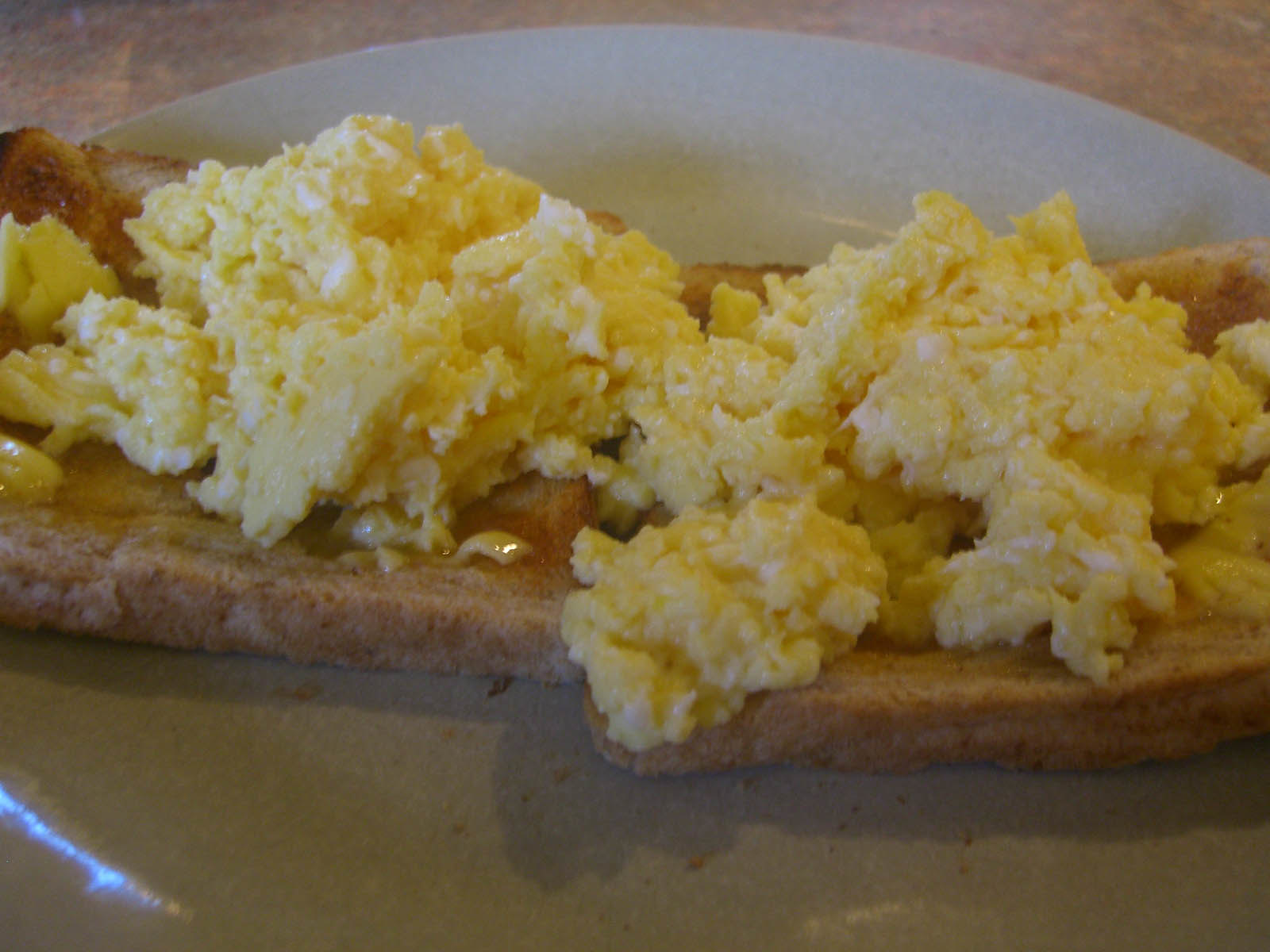The image is a close-up of a breakfast plate featuring scrambled eggs on whole wheat toast. The plate is a white round ceramic one, positioned on a beige or brown surface, likely a countertop or table. At the center of the plate are two square slices of toasted whole wheat bread, each topped with a generous mound of yellow, fluffy scrambled eggs. The toast appears crispy and a golden brown, with a slight buttery shine suggesting it has been buttered. The scrambled eggs, moist and slightly mushy, are heaped in a decent quantity, probably made from three or four eggs. A few crumbs are scattered around the toast, adding a subtle touch of authenticity to the image's homely setting.